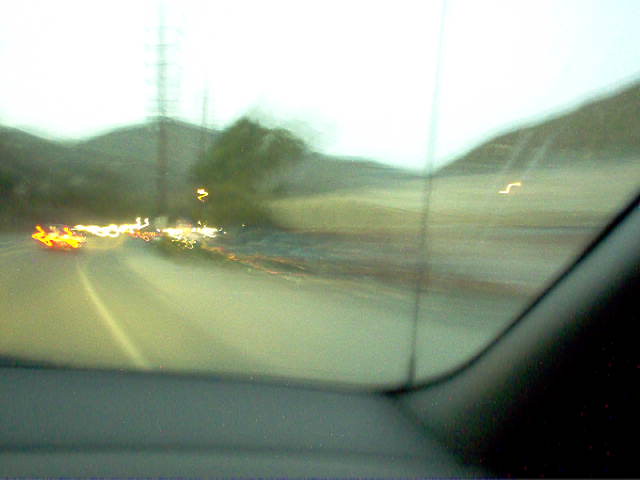This photograph captures a blurred view from the passenger seat of a moving vehicle on a freeway or highway. The interior, predominantly gray, includes part of the dashboard and an antenna visible through the window. Outside, there are hazy images of mountains or giant hills in the distance, interspersed with tall structures resembling power lines or telephone poles. A large tree stands to the right of these structures, next to what appears to be a field of grass or bushes. The foreground features a busy road with vehicles' headlights and taillights creating streaks of orange, yellow, and white in the motion blur, suggesting a lively scene with significant traffic. Additionally, a sidewalk or breakdown lane is discernible to the right side of the road. The entire scene, enveloped in a sense of movement, reflects the dynamic nature of travel and the landscape beyond.